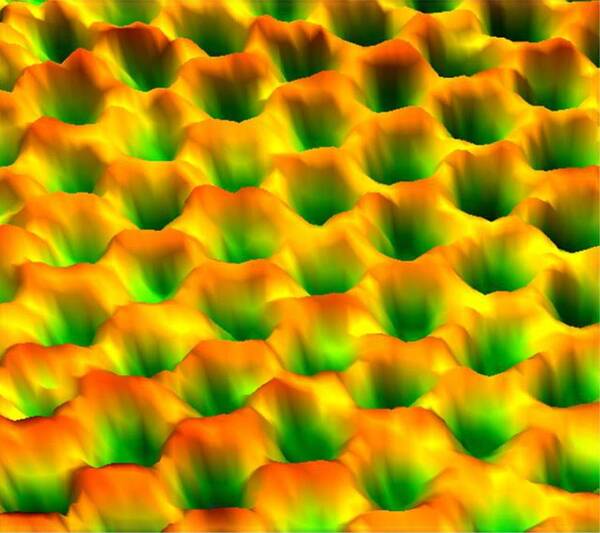The image features a highly detailed and vibrant repeating pattern that resembles a honeycomb or wasp nest. The structure consists of numerous circular or hexagonal indentations, creating a grid-like, lattice arrangement. At the bottom of each indentation, a fluorescent green color is prominent, transitioning upwards through gradients of light green, yellow, orange, and culminating in red at the tops. The pattern appears bumpy and mountainous, with deep ridges and valleys highlighted by the variation in colors. The overall effect is of a 3D, possibly computer-generated texture, although it also has a natural, organic appearance, making it difficult to distinguish if it is a natural or man-made object. The vivid colors and geometric consistency make it visually striking, with green being the dominant hue in the composition.